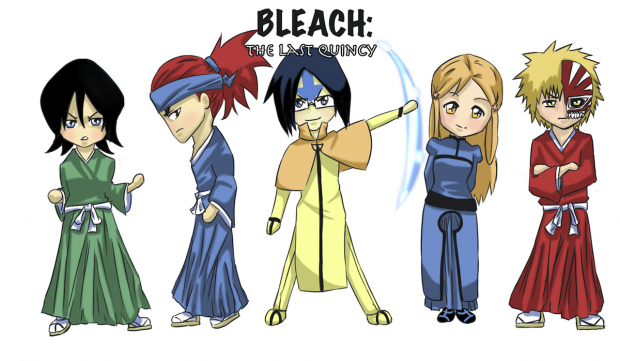This is an image featuring five anime characters from "Bleach: The Last Quincy." The background is pure white, allowing the characters to stand out prominently. Starting from the left, the first character is a woman with black hair wearing a green kimono. Next to her stands a man with bright red hair tied back with a blue headband and dressed in a blue kimono. In the center, there's a striking character, possibly male or female, with black hair and dressed in a yellow kimono, their left arm raised as if dodging or swinging. The fourth character, a woman with brown hair, is also in a blue kimono, actively dodging the central figure's movement. Lastly, on the far right, stands a man in a maroon kimono with frizzy yellow hair. Their distinct appearances are complemented by colors such as red, purple, yellow-green, brown, and white, creating a vibrant tableau under the black text at the top that reads "Bleach: The Last Quincy."